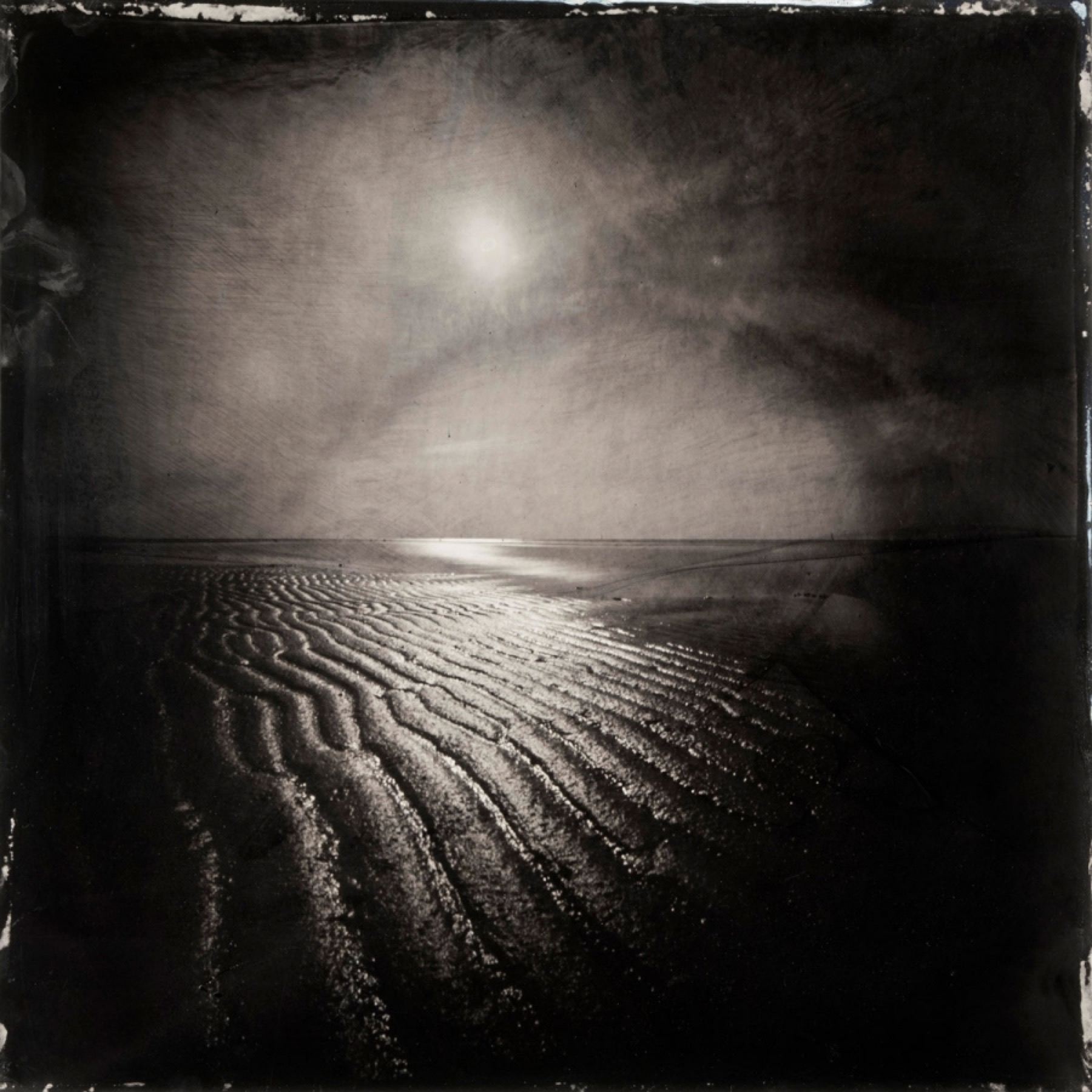The black and white image captures a mysterious, almost hauntingly beautiful beach scene. It appears to be a highly detailed charcoal sketch or created using dark ink, distinguished by its intense contrast. The composition is divided horizontally: the lower half features wet sand intricately detailed with rivulets and grooves formed by receding waves. This section exudes a sense of texture, showing where the water has flowed back into the ocean. The upper half of the image is dominated by a vast expanse of darkness, interrupted only by a faint, distant point of light—likely the moon or sun—shining through clouds. This light casts a delicate reflection on the water, adding a subtle glistening effect to the scene. The right side of the beach, just before it is swallowed by darkness, features a small, almost indistinguishable object. The image also shows signs of wear at the top edges, suggesting it's aged or well-handled, adding to its timeless and evocative character.